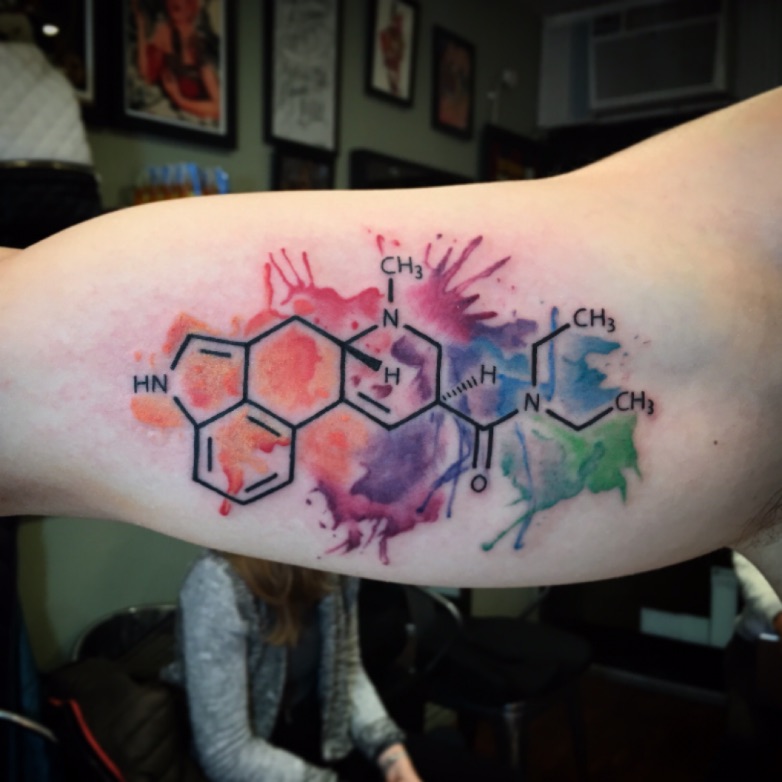The image features a colorful tattoo on the inner part of a white arm, depicting a complex chemical compound with elements such as hydrogen (H), nitrogen (N), carbon (C), and an oxygen (O) atom. The compound includes three carbon atoms, several hydrogen atoms in different configurations (HN, CH3, HHNCH3), and splashes of vibrant colors ranging from peach-red to purple, blue, and green form the background. In the dimly lit tattoo parlor, a wall adorned with various pictures and frames can be seen. A woman with white skin, wearing a gray jacket and seated on a black chair with a black backpack beside her, is visible, though slightly blurred in the background. The focus of the lighting in the image emphasizes the detailed and colorful tattoo on the bicep, while the background remains subdued.